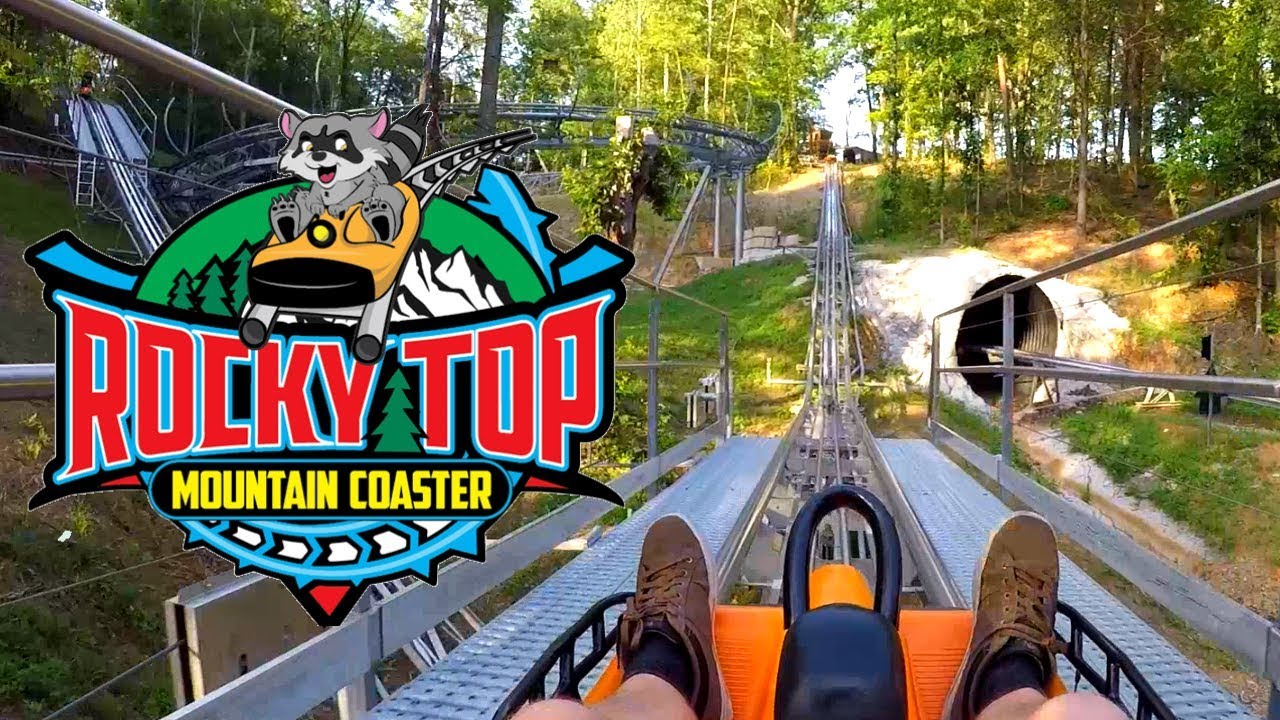The image is an advertisement for the Texas Reeds Rocky Top Mountain Coaster and prominently features vibrant scenes from an amusement park set against a lush forest backdrop. On the left side of the image, a circular logo in red and yellow announces "Rocky Top Mountain Coaster," with a playful illustration of a raccoon riding a yellow roller coaster. Below the logo, the actual roller coaster is visible, winding its way through dense trees and emerging from a tunnel that interestingly looks like a drain pipe.

Dominating the foreground, a POV shot shows a young man with brown tennis shoes and black socks riding an orange coaster cart, poised on a straightaway section of the track before heading uphill. The coaster tracks weave in and out of the forest, crisscrossing and overlapping. To the left of the man, another section of track dips downward, suggesting the possibility of multiple interconnected roller coaster paths. This seamless blend of thrilling coaster design with natural surroundings makes it clear that the Rocky Top Mountain Coaster offers a unique ride experience, combining the exhilaration of roller coaster drops and turns with the beauty of a forested mountain.